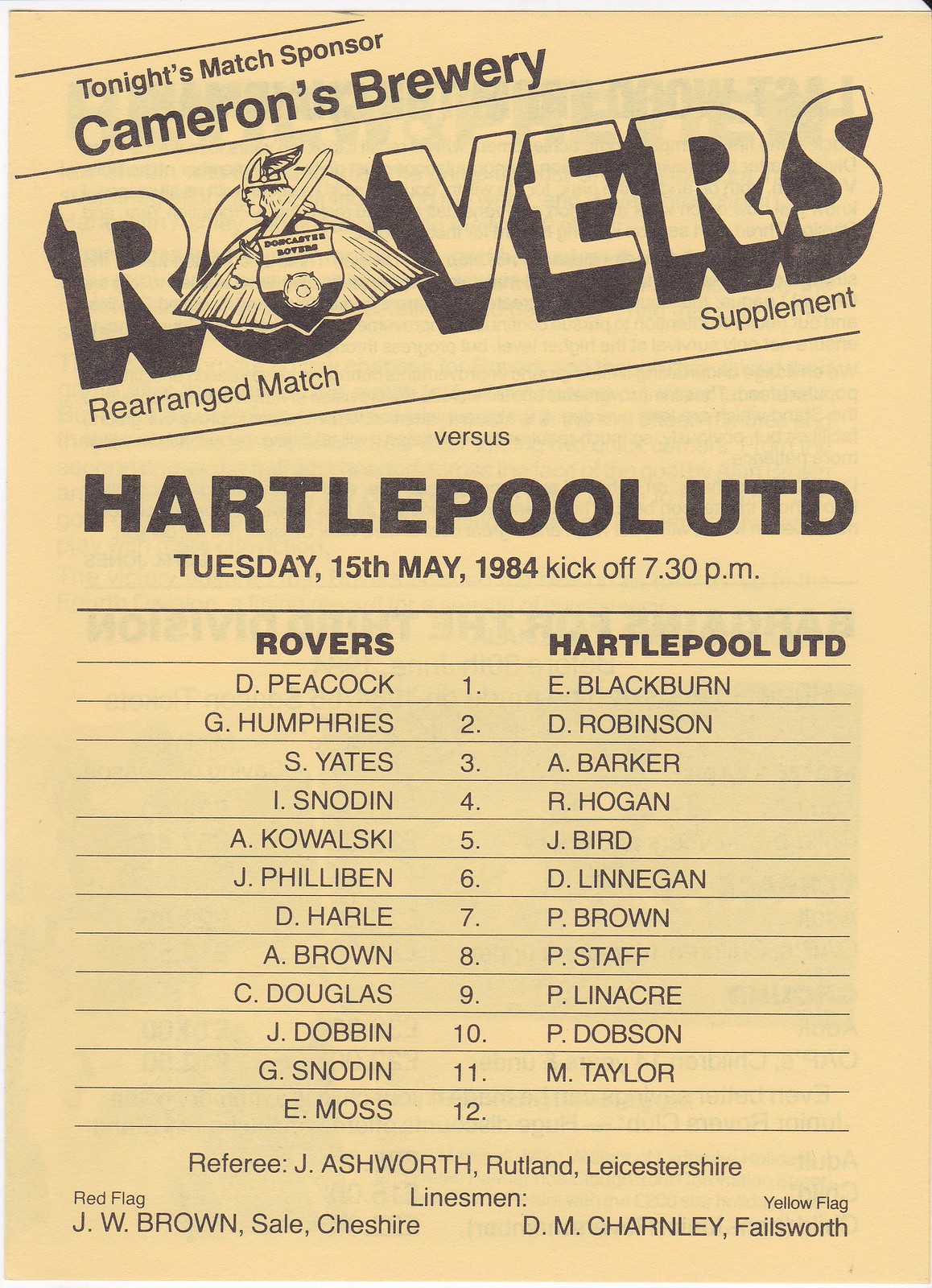The image is a yellowing advertisement paper featuring details of a football match. The text is black and the layout is slightly diagonal from the bottom left to the upper right. At the top, it reads "Tonight's Match Sponsor" in black text, followed by a larger black text "Cameras Brewery." Below a black dividing line, the largest text "Rovers" appears, with a slight 3D effect on the black-edged letters. The 'O' in "Rovers" contains a logo of a Viking facing left, wielding a sword over his shoulder and a shield facing forward. Beneath, it says "Rearrange Match Supplement," followed by another dividing line with the word "Versus" in black text, then "Hartlepool UTD" in bold black text. The match details are listed below: "Tuesday, 15th May 1984, Kickoff 7:30 p.m." The paper includes the lineup for both teams: Rovers have 12 players, Hartlepool UTD has 11 players. Below the lineups, it mentions the match officials: Referee J. Ashworth (Rutland), Linesmen: Red flag J.W. Brown (Cheshire) and Yellow flag D.M. Charles (A. Fellsworth).